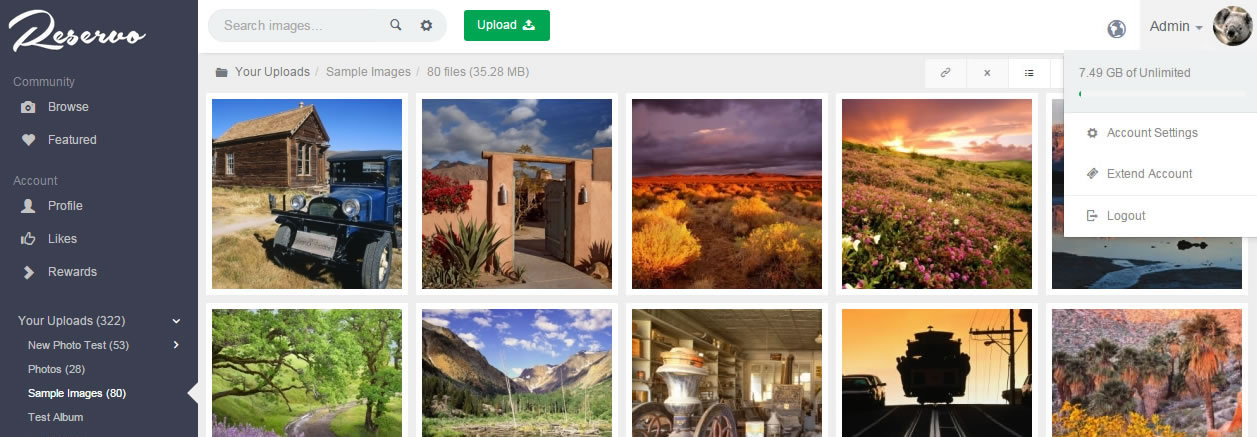The image features the interface of an application named Reservo. On the left side, a sidebar displays various menu options labeled as follows: Community, Browse, Featured, Account, Profile, Likes, Rewards, Your Uploads (322), New Photo Test (53), Photos (28), Sample Images (80), and Test Album. 

To the right of the sidebar is a search bar with the placeholder text "Search Images." The search bar is accompanied by a magnifying glass icon and a settings gear icon. Further to the right, there is a globe icon followed by the label "Admin," alongside a profile picture that appears to be a small image of either a sloth or a koala. Below this, the account status reads "7.49 GB of Unlimited," highlighting the storage used. 

Additional options below the account status include "Account Settings," "Extend Account," and at the bottom of the sidebar, "Logout." 

In the main section of the interface, there are 10 images displayed, predominantly showcasing outdoor nature scenes. The images are arranged with five or more in a visible row, emphasizing the visual aspect of the platform.